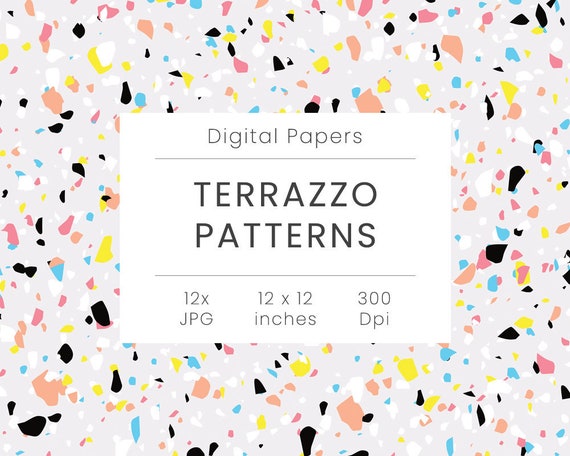This is a square graphic displaying an advertisement or packaging for digital papers. At the center of the graphic is a white rectangle with black text reading "Digital Papers" prominently in bold. Below, it states "Terrazzo Patterns" and details such as "12 JPG," "12 by 12 inches," and "300 DPI." Surrounding the white rectangle is a border decorated with jagged, confetti-like fragments in colors including pink, black, blue, yellow, white, and orange, creating a playful terrazzo pattern. The background of the graphic is a light gray, enhancing the vibrant fragments. The design suggests the product consists of high-resolution digital papers with terrazzo patterns, suitable for various creative projects.